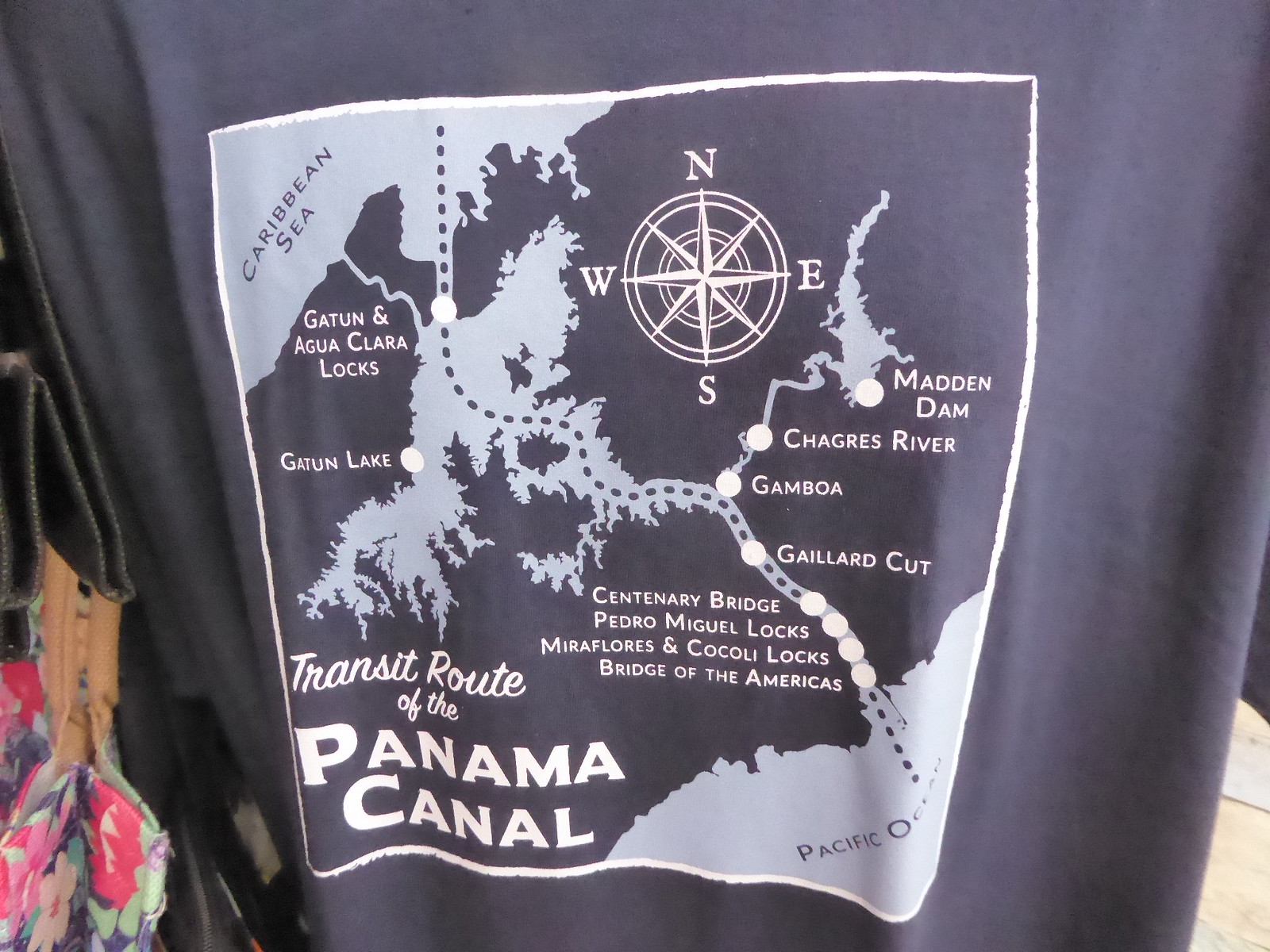This image features a dark blue t-shirt that prominently displays a detailed map highlighting the transit route of the Panama Canal. The design showcases a light blue map overlaid with white text, depicting the intricate waterways and landmarks of the canal. A nautical compass adorns the top middle of the map, indicating the north, south, east, and west directions. The map features a dotted line, marking the route through various significant points, including the Caribbean Sea, Gatun and Agua Clara Locks, Gatun Lake, Madden Dam, Chagres River, Gamboa, Gaillard Cut, Sanitary Bridge, Pedro Miguel Locks, Miraflores and Cocoli Locks, and the Bridge of the Americas, culminating at the Pacific Ocean. The bottom left of the design bears the caption "Transit Route of the Panama Canal," encapsulating the tourist-centric nature of the shirt and offering a thorough guide through the famed canal's passageways.